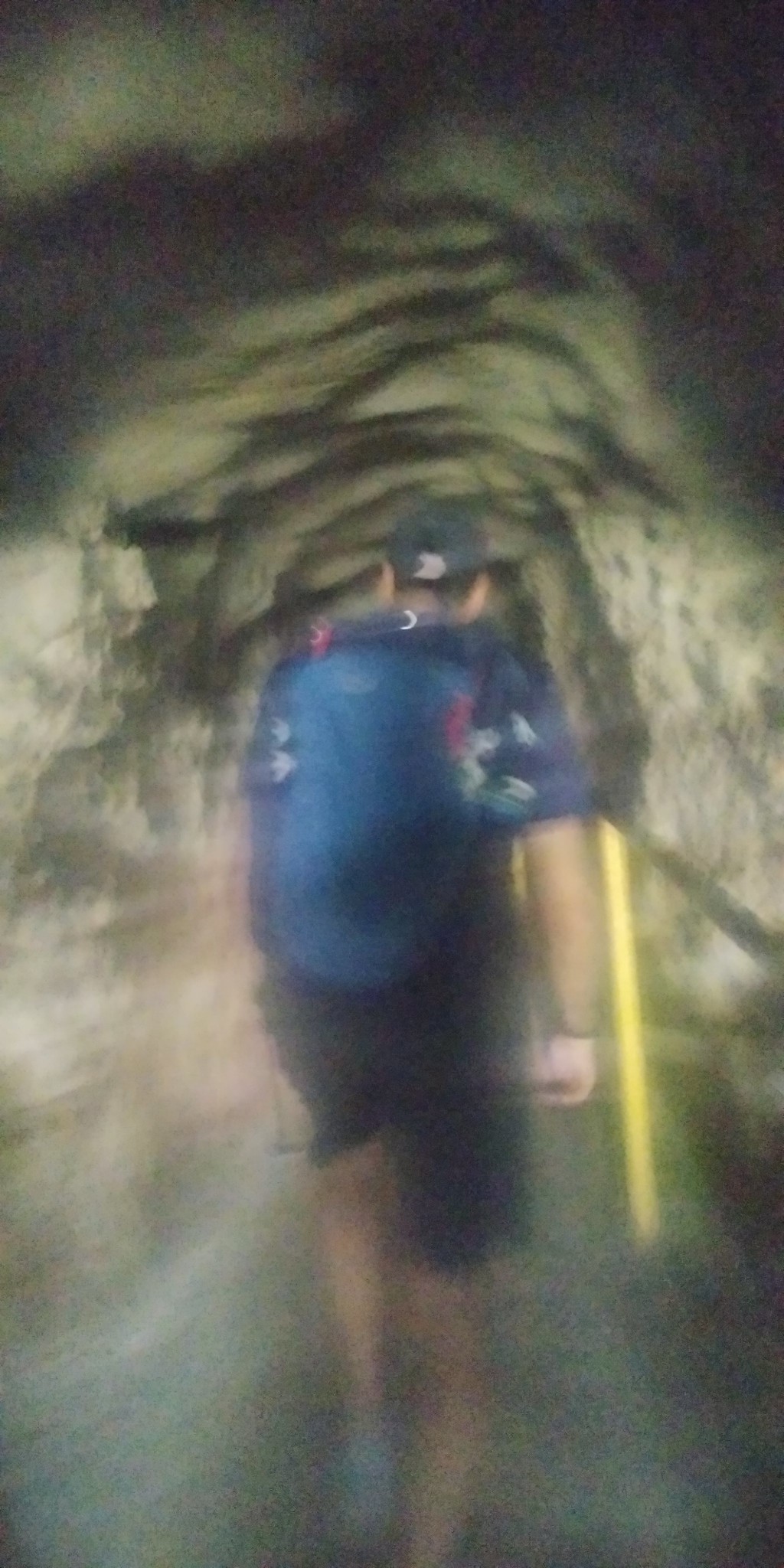A highly artistic and intentionally blurred rectangular portrait-oriented photograph captures the back of a man walking away in what appears to be a cave. The Caucasian man is dressed in dark blue shorts, a blue short-sleeved shirt, and a grayish-blue cap, revealing his ears and dark hair. A blue backpack is slung over his shoulders, and something adorns his right wrist. As he walks, his relaxed arms hang by his sides. The cave environment is dimly lit, with darker shadows above and a visible path curving into the distance. To the man's right, a vertical yellow guide rail stands out against the natural tones of the cave, providing a stark, almost surreal contrast to the scene.